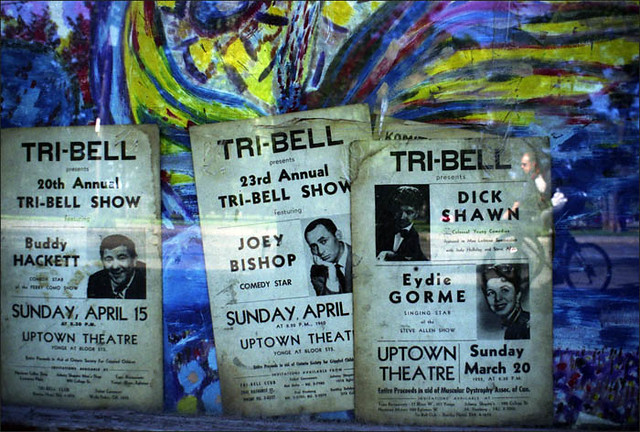The image depicts a vibrant, colorful wall that features an abstract design with swirling patterns in shades of blue, green, yellow, and red. Toward the bottom of the artwork, the abstract elements give way to more recognizable shapes, including white flowers with yellow centers and what appears to be an audience. Overlaid onto this painted surface are three vintage handbills or flyers, seemingly taped to a glass window or reflection surface. The handbills are for Broadway-style shows at the Uptown Theatre, featuring 1950s comedians. The top flyer reads "Tribell presents the 20th annual Tribell show featuring Buddy Hackett, Sunday, April 15th." The middle flyer advertises "Tribell's 23rd annual Tribell show with comedy star Joey Bishop, Sunday, April," though the exact date is obscured. The third flyer mentions "Tribell, Dick Shawn, Edie Gourmet, Uptown Theatre, Sunday, March 20th." The reflective surface creates a layered effect, where the colorful wall, the handbills, and the faint reflections of a bicyclist and a car are all visible, adding depth to the scene.